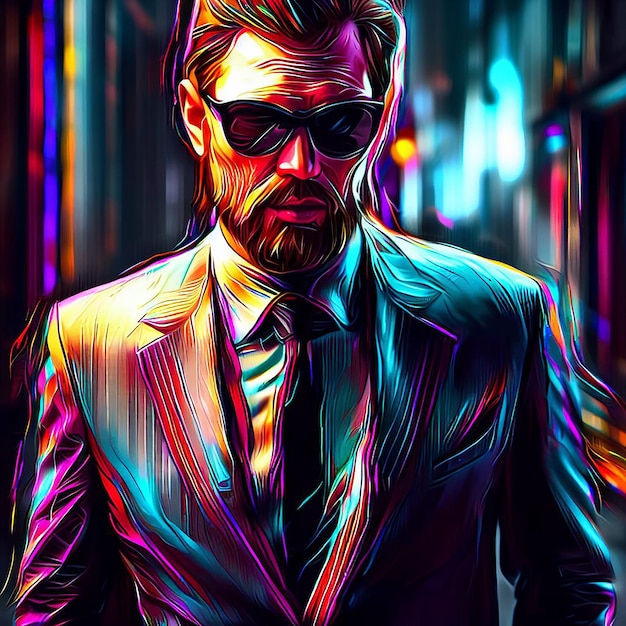The digital image portrays a vibrant, psychedelic depiction of a Caucasian man resembling John Wick, dressed in a suit and tie. The man features long, dark, slightly slicked-back hair and wears dark sunglasses over a face marked with wrinkles and adorned with a goatee. The image primarily uses a spectrum of bright, neon colors, including blue, pink, purple, red, yellow, black, brown, and teal, which blend seamlessly throughout the scene. The background appears blurry, obscuring specific details but maintaining the overall vivid color scheme. The man is centered in the composition, viewed from the waist up, with the knot of his tie also centrally positioned. The overall aesthetic gives the impression of an AI-generated, psychedelic artwork, rich in color and dynamic in style.